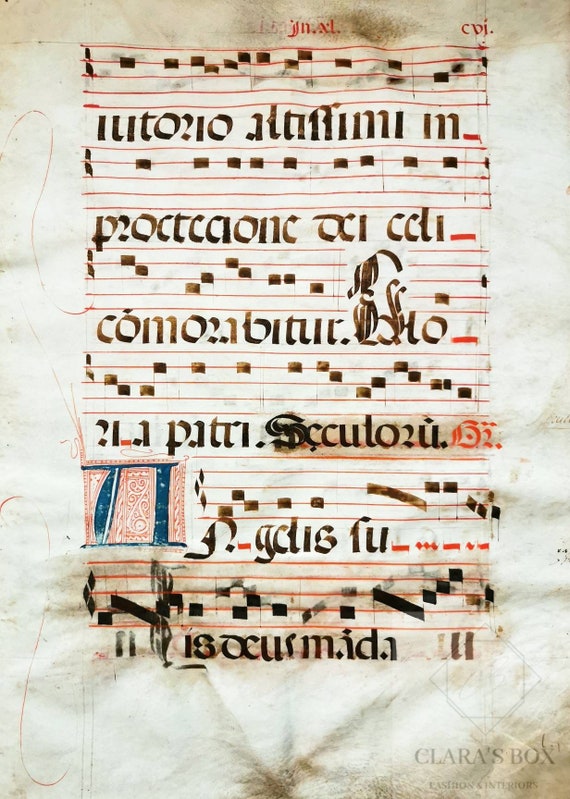This vertical rectangular image features an ancient, weathered piece of sheet music printed on white paper that has aged into shades of yellow, brown, and blackish tinges at the top. The sheet music displays rows of red lines, presumably music bars, with square-shaped notes lacking tails. Black rectangular notes are present on these lines, and the lines often appear faintly or with alterations and additions through the piece. Underneath the notes, there are lines of text that seem to be written in Latin, accompanied by various markings hinting at either musical or instructional notations. The text itself appears calligraphic in style. At the bottom left, a distinct decorative symbol akin to the pi symbol in blue, framed by a red carving-like background, can be seen. Towards the bottom right, a watermark reading 'Clara's Box' along with something indicating 'Interiors Easton' is visible.